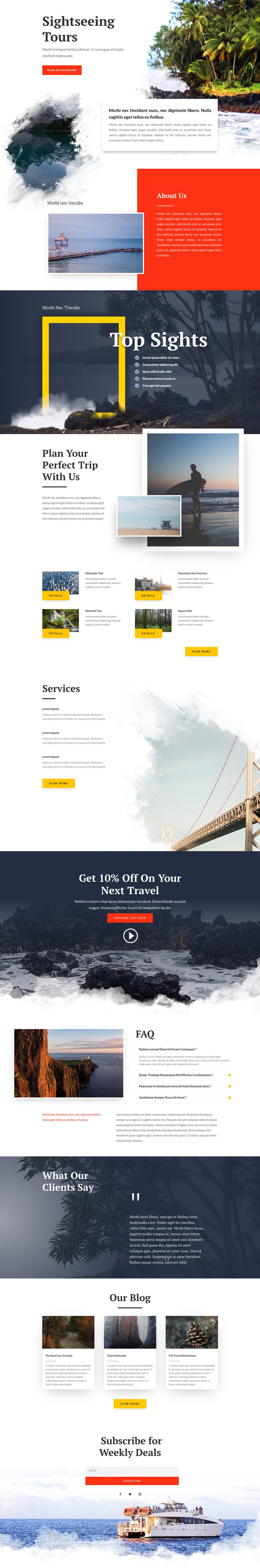This color image is in a portrait format, depicting a series of National Geographic online pages captured in screenshots. The screenshots are arranged vertically, creating the appearance of one continuous page. The text on the page is very small, making it challenging to read on a smartphone without substantial zooming. The content doesn't seem formatted for easy viewing on a smaller screen, suggesting it might be from a desktop or laptop view.

The title at the top of the page reads "The Top Sightseeing Tours." Below this, there is a list of top sights, though the small text size renders the specifics unreadable. The page features a mix of textual content and vibrant photographs, displaying a variety of breathtaking locations. These images include a tropical area with a beach, a person surfing, a picturesque bridge, a mountainous landscape, possible glaciers, and a lovely catamaran boat. The composition of the images and text aims to showcase diverse and exciting travel destinations.